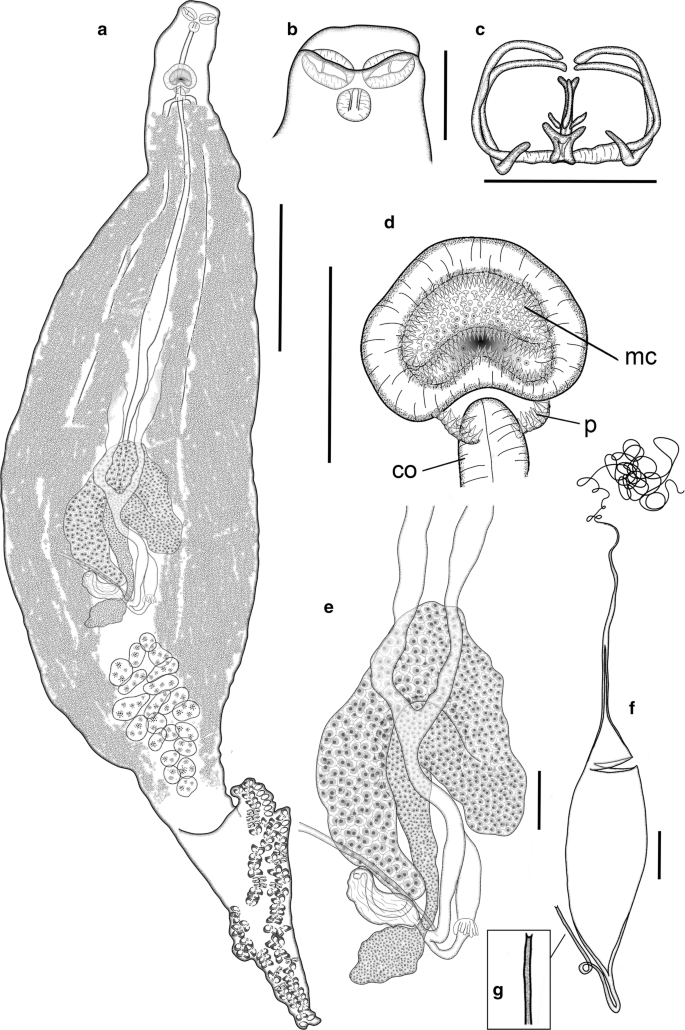The image features a detailed black and white diagram of various anatomical parts, each labeled with letters from A to G. Starting on the left, a long, cylindrical shape labeled A extends from the top to the bottom, resembling a yam with internal squiggles and round elements, suggestive of a stomach. Diagram B, a curved line with internal ovals, is next. Moving to diagram C, it depicts a structure that looks akin to a uterus with what could be Fallopian tubes. Diagram D shows a rounded section containing smaller cells labeled MCP, P, and CO, potentially similar to brain tissue. Below D, diagram E appears as a mass of squiggly organ-like shapes. Diagram F features a lengthy object with a squiggly line, reminiscent of sperm, and next to it, an enlarged section labeled G. The entire illustration, done in shades of gray with black outlines, showcases various shapes and forms that seem to represent an eclectic mix of anatomical organs or structures.